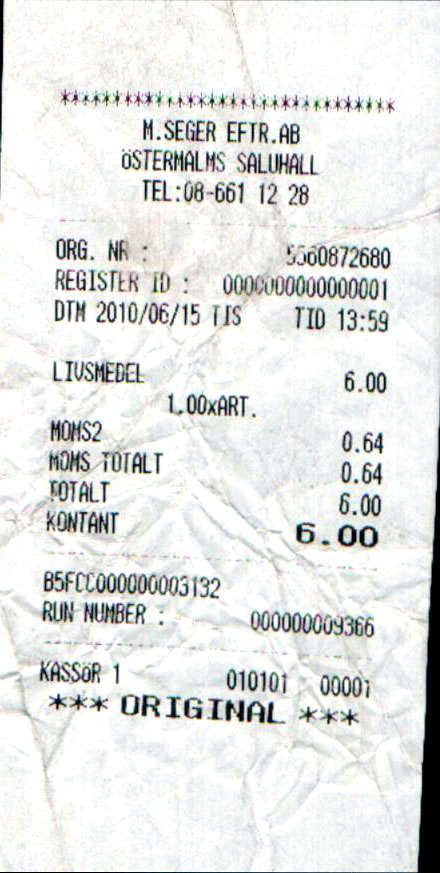A crumpled and then smoothed-out, long rectangular shopping receipt on white paper. The black text is visible despite the wrinkles. At the top center, a row of stars spans from right to left. Below the stars, the header reads "M. Seger, F.E.F.T.R. A.B. Ostermalms, Saul Hall, Saul U. Hall," with the telephone number "08-661-1228" underneath. Further down, an "O.R.G. N.R." label is partially obscured by a blur, followed by a sequence of numbers. There is also a "Mr. I.D." section with a string of mostly zeroed numbers. The receipt lists items totaling 64 cents, culminating in a final amount of six dollars. The word "original" is printed at the very bottom.